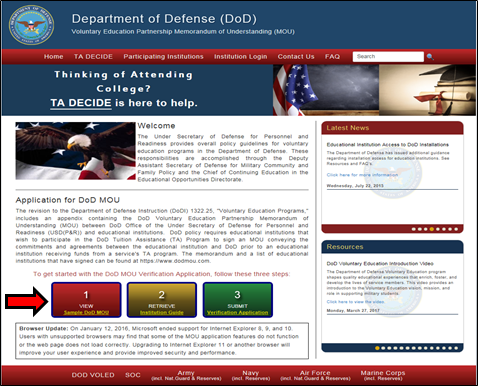The image depicts an official website for the Department of Defense (DOD), specifically focusing on the Voluntary Education Partnership Memorandum of Understanding (MOU). At the top of the webpage, the header clearly states "Department of Defense (DOD) Voluntary Education Partnership Memorandum of Understanding (MOU)," accompanied by a circular icon featuring an American eagle.

Below the header, there is a prominent red navigation bar with menu options including Home, TA Decide, Participating Institution, Institution Login, Contact Us, FAQ, and a search box. Under this bar, a banner reads "Thinking of Attending College? TA Decide is here to help," displayed alongside an image of books, a diploma, a graduation cap, and a chalkboard.

The main content section introduces with a welcome message: "The Under Secretary of Defense for Personnel and Readiness provides overall policy guidelines for voluntary education programs within the Department of Defense. These responsibilities are executed through the Deputy Assistant Secretary of Defense for Military Community and Family Policy, and the Chief of Continuing Education and Educational Opportunities."

To the right, there's a "Latest News" section highlighted with a red header, followed by another section labeled "Resources." Underneath the welcome message, a notice about the revision to the Department of Defense Instruction (DODI) 1322.25 is posted, along with an application for the DOD MOU.

Further down, there are three colorful boxes—red, yellow, and green—detailing steps to get started with the DOD MOU verification application: Step 1: View, Step 2: Retrieve, and Step 3: Submit. Each step is emphasized by a red arrow and yellow links beneath the instructions.

At the bottom of the page, another red bar lists various military branches: DOD, VOLED, SOC, Army, Navy, Air Force, and Marine Corps. There is also a section labeled "Browser Update."

The detailed layout provides clear guidance and numerous resources for individuals interested in participating in the DOD voluntary education programs.